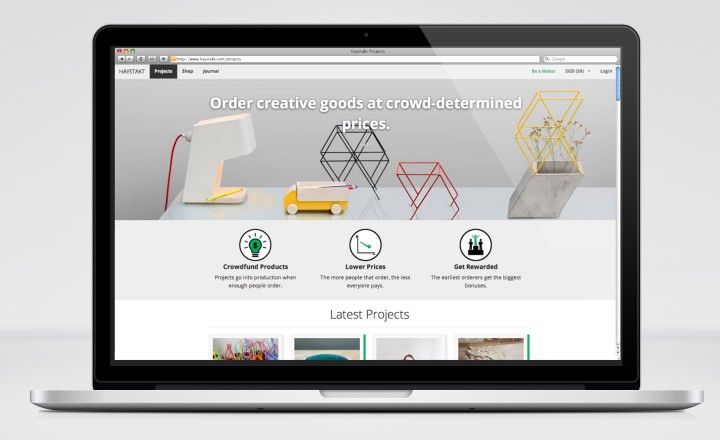The image depicts a laptop or tablet with a black exterior, displaying a website on its screen. At the center of the screen, the text reads: "Order creative goods at crowd-determined prices." The scene is set on a white table adorned with various geometric shapes.

On the far right, there is a silver geometric pot holding a small plant with tiny flower buds, topped with a yellow geometric wire design. To its left, there is a red geometric design followed by a black geometric piece resembling a Ferris wheel. Continuing leftward, there is a yellow toy truck with a white bed, which appears to contain a crayon. The truck has white tires. Further left, there is a small white machine emitting light from its bottom, with a red cord attached on the left side.

In the upper left corner of the laptop screen, some colored icons in red, yellow, and green are visible, although they are blurry. Below these icons, three descriptive circles provide information about the website's offerings: 

- The first white circle with a black border features a green light bulb with a dollar sign, and below it, the text reads: "Crowdfund products. Products go into production when enough people order."
- The second circle highlights: "Lower prices. The more people that order, the less everyone pays."
- The final circle emphasizes rewards with the text: "Get rewarded."

The overall scene is a mix of digital and physical elements, focusing on promoting the website's unique approach to shopping.